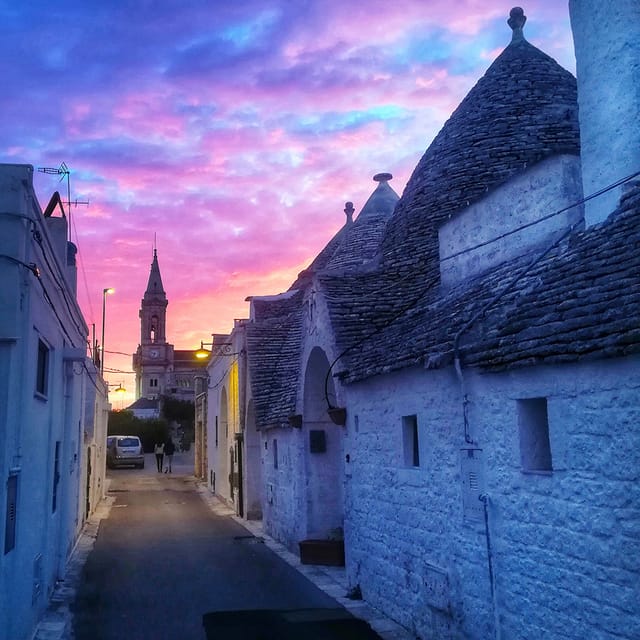In this captivating square photograph, the setting sun creates a stunning display of colors, transitioning from deep blues and purples at the top of the sky to vibrant pinks and a golden orange near the horizon. This remarkable sunset illuminates a narrow alley or street in an ancient village, characterized by white stone buildings on either side. These structures, with their rough-hewn bricks and small square windows, are topped with dark gray or black slate roofs, some adorned with domes. The right side of the alley features two prominent archways, while one streetlight casts a gentle glow on a doorway below.

The serene street is devoid of trees, instead lined with these quaint, individual-height buildings that appear to be single-storied. At the far end of the alleyway, a tall church steeple and a clock tower rise into the dusky sky, partially obscured by power lines threading through the scene. Streetlights have already come to life, their warm light mingling with the last rays of the sun.

In the distant background, two tiny figures can be seen near a parked car, adding a touch of life to this tranquil snapshot of timeless architecture and breathtaking natural beauty.